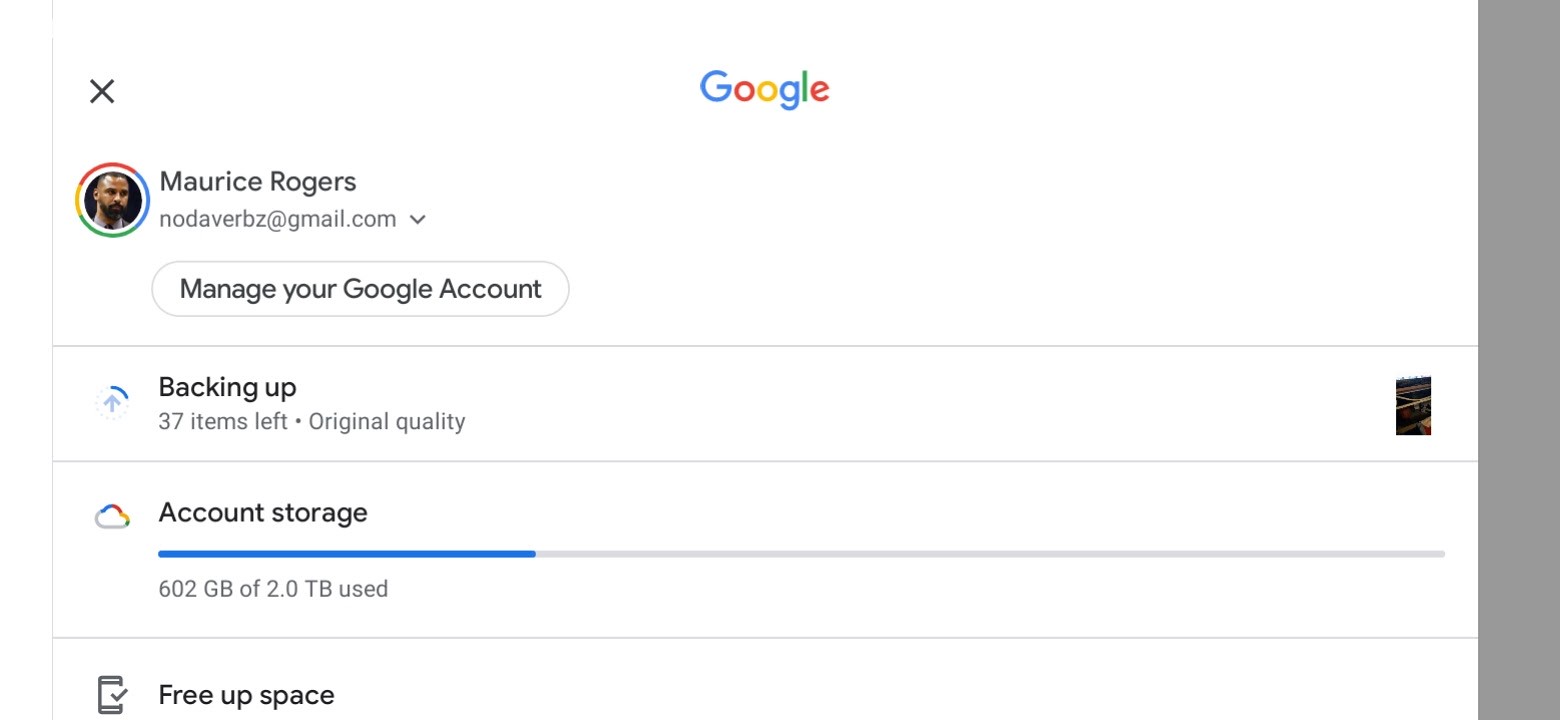The image appears to be a screenshot of a Google account management interface. At the top, the word "Google" is displayed in its traditional multi-colored logo. In the upper right corner, there is an 'X' icon for closing the screen. Below the Google logo, there's a small circular profile picture, accompanied by the name "Maurice Rogers." Adjacent to the name is the email address "notoverbs@gmail.com."

Underneath this section, within an oval outline, there is a button labeled "Manage your Google Account." A horizontal grey line spans the width of the screen, separating the top section from the subsequent information.

The next section indicates the backup status, reading "Backing up - 37 aisles left - Original quality." On the far right of this line, there is an indiscernible black rectangle.

Another thin grey line separates the previous section from the next one, which is labeled "Account storage." This section includes a blue progress bar, approximately one-fourth of the way filled, indicating storage usage. Below the progress bar, it states "602 GB of 2.0 TB used."

Another thin grey line follows, under which there's a "Free up space" option. All text, aside from the colorful Google logo, is in black. On the far right side of the screen, there is a tall, narrow grey rectangle that extends from the top to the bottom.